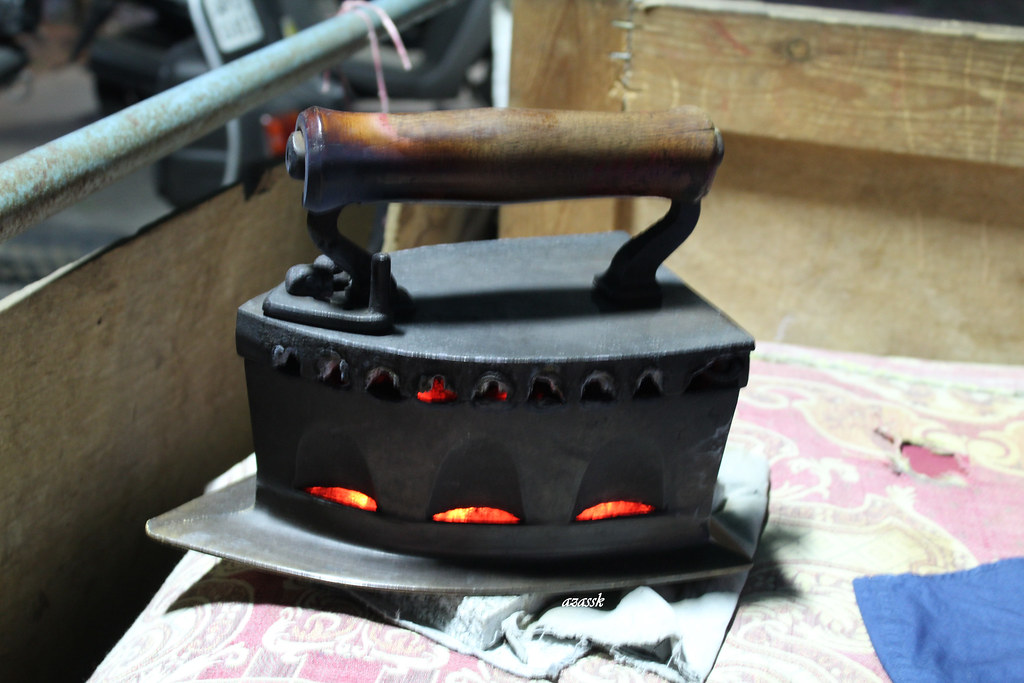This landscape-oriented color photograph showcases an antique coal iron with a worn, slightly scorched wooden handle. The iron has a sturdy, dark gray iron body with a shield-shaped soleplate, displaying an old-fashioned design. The side walls of the iron feature three slits, through which glowing, red-hot coals can be seen. The iron is centrally placed atop a rolled-up segment of white cloth, pressing it down. This white cloth rests on a pink piece of fabric, beneath which a red cloth is partially visible. In the bottom right corner, there is a small piece of blue fabric. The scene is brightly lit by daylight, highlighting the antique iron against an outdoor backdrop that includes a fence or short wall with a railing to the left. The photograph embodies the style of photographic representationalism realism.